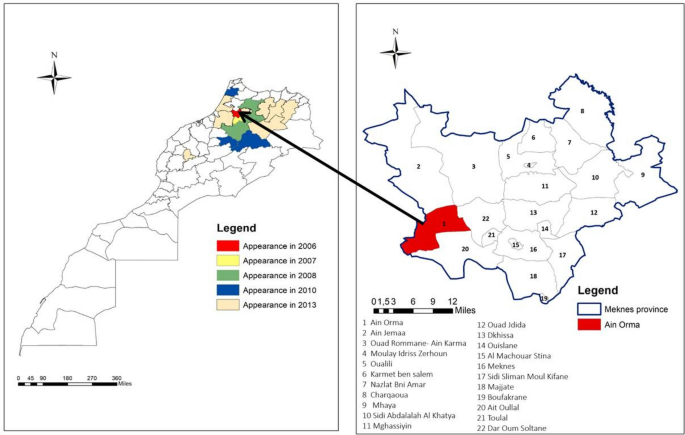The image depicts two distinct maps drawn on separate pieces of paper, placed side-by-side with a slight gap in between. Each map is enclosed by a thin black pinstripe outline. Combined, the maps measure approximately 5 inches in width and 3 inches in height. 

The map on the left displays a detailed, color-coded representation of a larger portion of a country, featuring a variety of colors corresponding to different years: red for 2006, yellow for 2007, green for 2008, blue for 2010, and tan for 2013. This map includes a legend located below that explains these color codes. A four-pointed compass star with an 'N' at the top indicates the north direction, situated at the upper left corner. Additionally, there is a scale at the bottom left corner indicating a distance of 0 to 300 miles.

On the right-hand map, a focused segment of the country is shown, highlighting only one section colored in red, labeled as section number 4 from the year 2006. Below this map, the legend details the broader area names and their respective numbers from 1 to 22, which are marked on the map. The white areas are indicated to be the Meknes province and a small orange region named Ain Orma. This map also includes a compass star with an 'N' and a different scale, ranging from 0 to 12 miles. An arrow points from this detailed map to the corresponding red area on the left map, illustrating the zoomed-in view of that specific location.